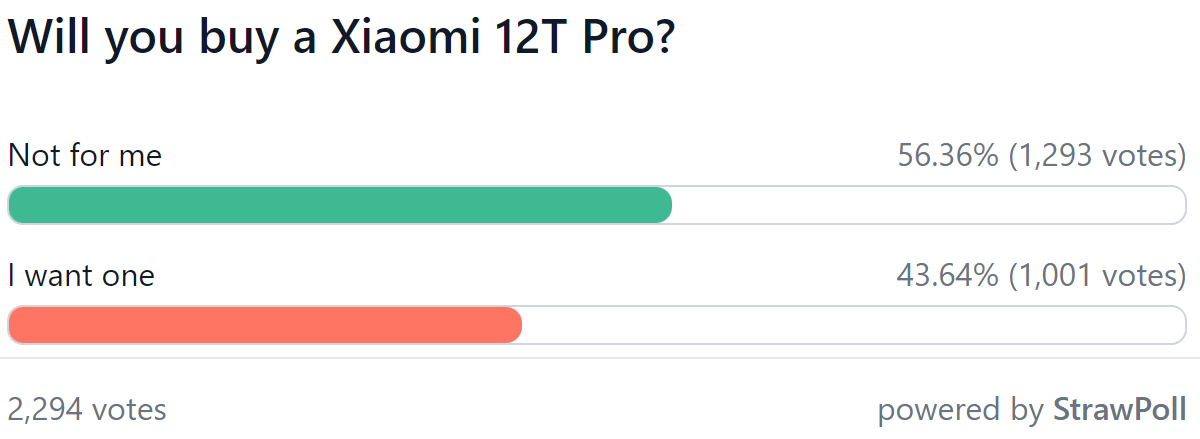In this image, a poll is depicted regarding the potential purchase of a Xiaomi 12T Pro. The poll results are visualized with two distinct colored ovals. The green oval, representing the option "Not for me," indicates that 56.36% of respondents (1,293 votes) are not interested in buying the phone. The red oval, which signifies the option "I want one," shows that 43.64% of participants (1,001 votes) are willing to purchase the device. The total number of votes cast in this poll is 2,294. At the bottom left of the image, it is mentioned that the data is powered by a robust bubble chart, illustrating a strong visual representation of the polling outcome.